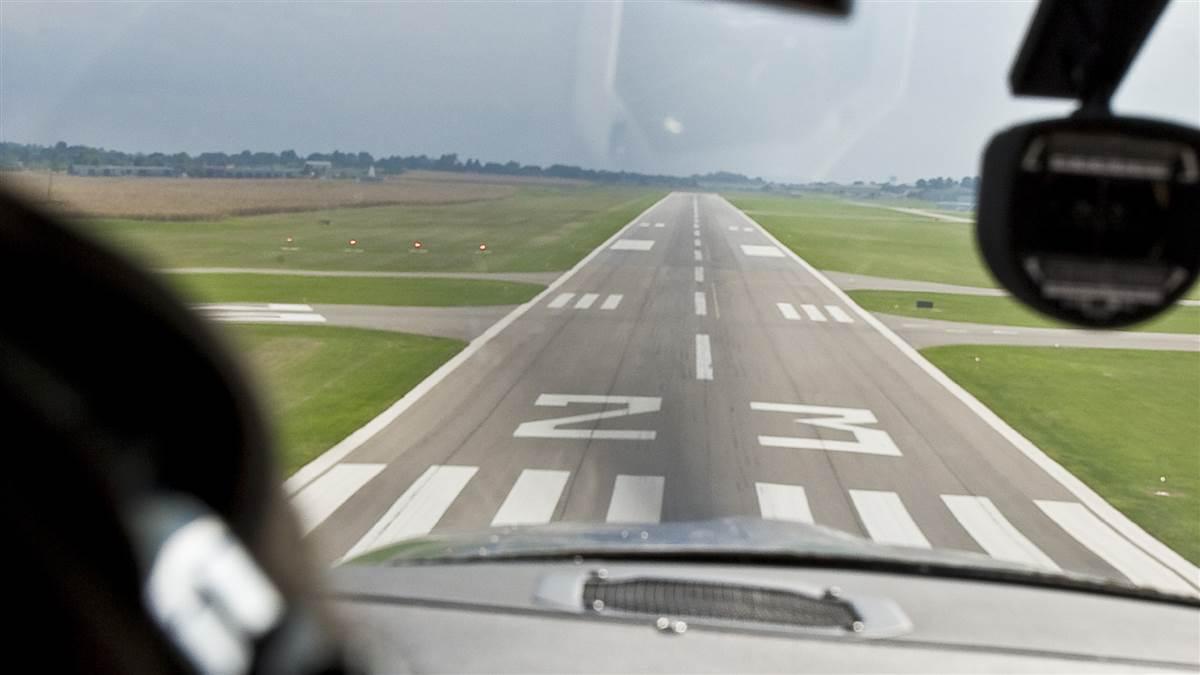The image captures the view from the cockpit of a plane or helicopter, looking out through a window at a runway. The expansive landing strip stretches from the bottom corners of the image and narrows towards the horizon, which is about a quarter of the way down the image. The sky above is gray, providing a muted backdrop. Flanking the runway are vast, green fields with some scattered trees, and faint outlines of smaller roads branching off to each side.

The runway itself is a smooth, dark surface, with a sequence of white lines. A dashed line runs down the center, flanked by solid lines on either side. Toward the foreground, the runway is marked with the number "23" and features a series of transverse lines. To the top right of the image, an unreadable gauge is mounted, and at the bottom, part of the aircraft's dark dashboard with a vent is visible. Additionally, the image includes the back of the pilot's head wearing a headset on the left, and a glimpse of the plane or helicopter's nose at the bottom.